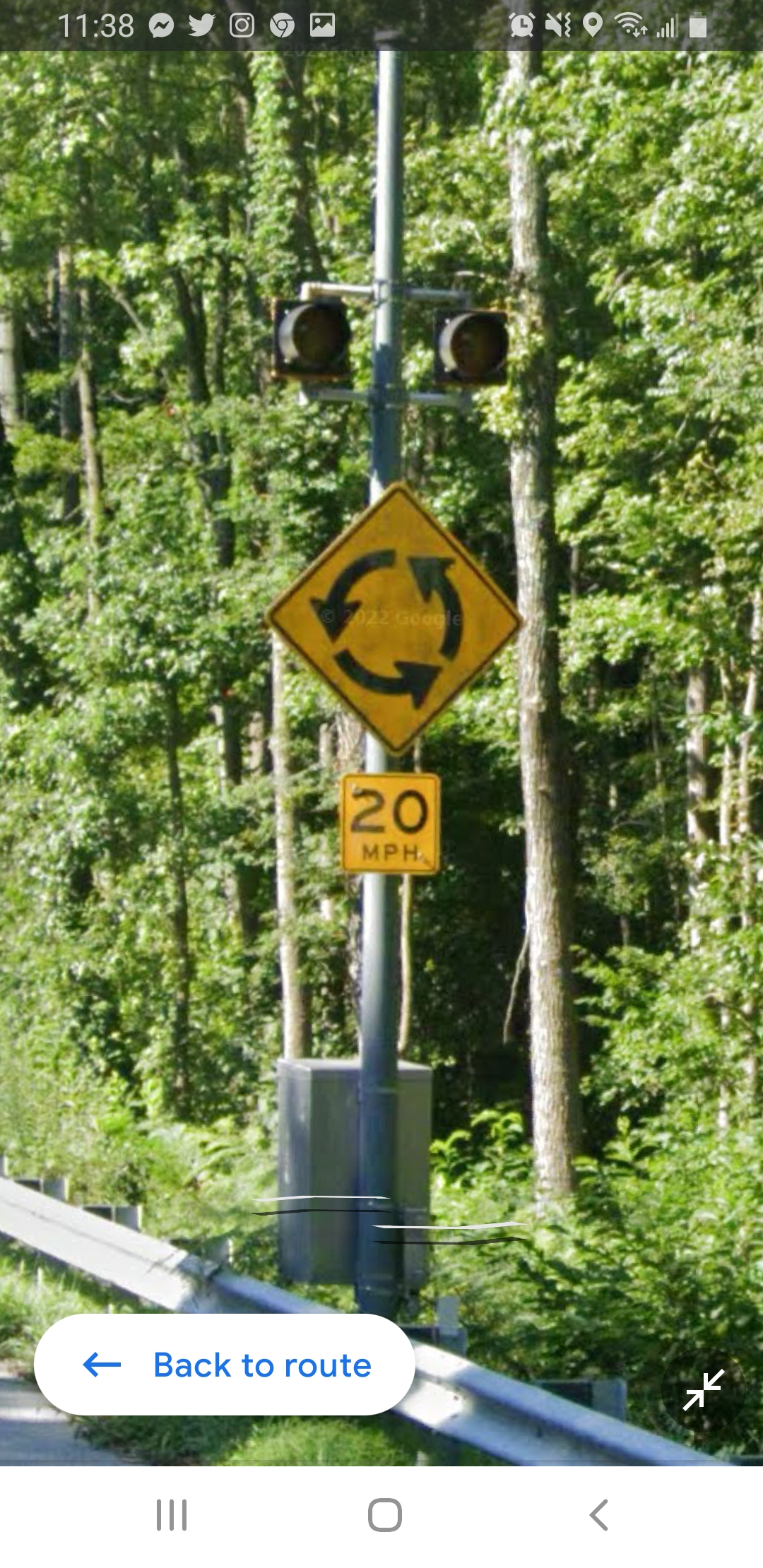This detailed photograph captures a computer screen displaying an outdoor scene. The top edge of the screen features a black border with the time "11:38" displayed in white text. The screen also shows a variety of icons, including the familiar bird logo indicating the presence of the Twitter app, a sound icon, a Wi-Fi signal indicator, and a fully charged battery icon.

The central image on the screen is a vibrant outdoor scene dominated by lush green trees. Prominently in the foreground stands a metal pole supporting a diamond-shaped, yellow caution road sign. This sign features three black arrows arranged in a circular pattern, and it specifies a speed limit of 20 miles per hour. Additionally, the sign includes a small white banner at the bottom, displaying the text "Back to Route" in blue letters, along with a left-pointing arrow.